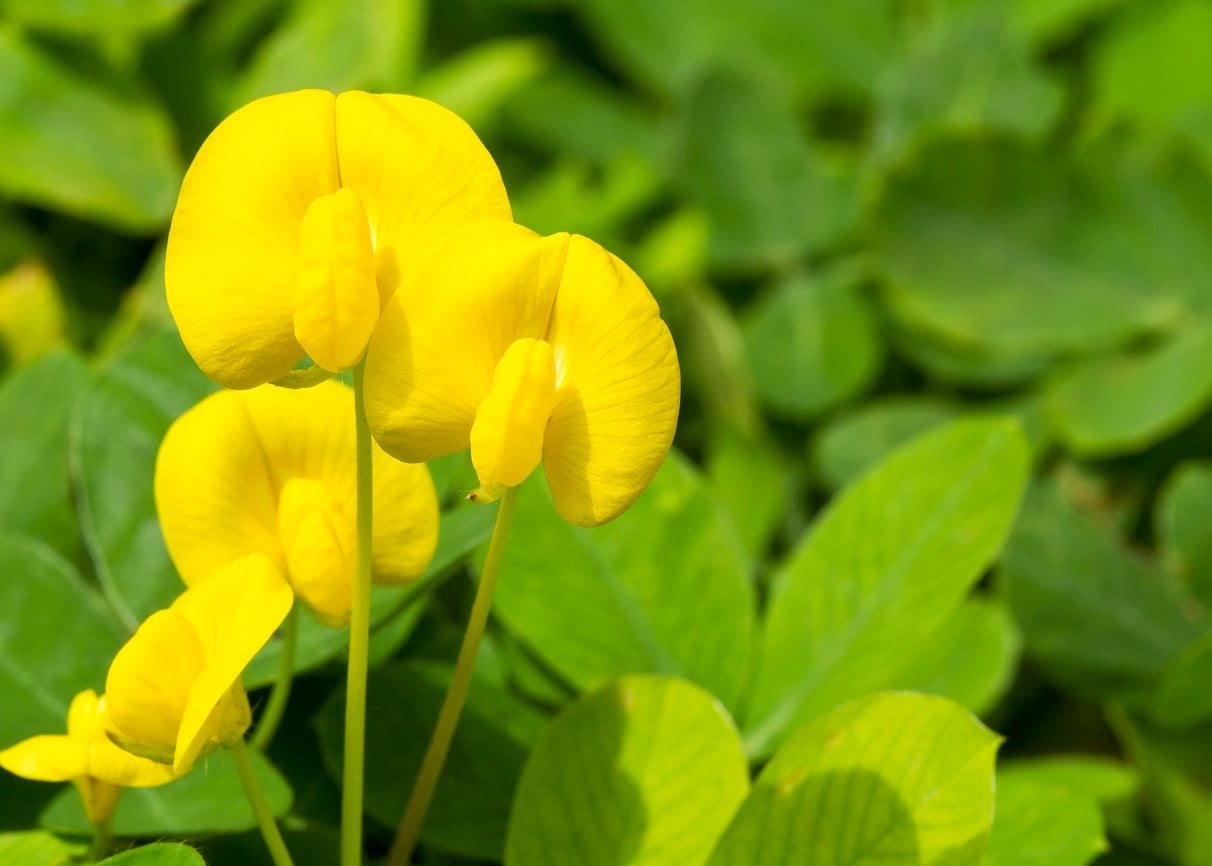This close-up color photograph captures a vibrant cluster of yellow flowers amidst lush green foliage, suggesting a bright sunny day. The background is slightly blurred, highlighting a strong depth of field effect, and comprises a variety of green stems and leaves in shadows, giving the scene a rich, textured look. The foreground, positioned slightly to the left, features four to five yellow flowers at different stages of blooming. The flowers are atop long green stems, with one flower only partially open at the bottom left, followed by middle ones in various stages of flowering, and the topmost flowers are fully open. Each flower has a distinctive appearance with wide, rounded yellow petals and what appears to be a central, pillow-like structure of the same material. The perspective appears elevated yet close, allowing a detailed view of the flowers which are small in size, adding to the intimate feel of the nature scene.